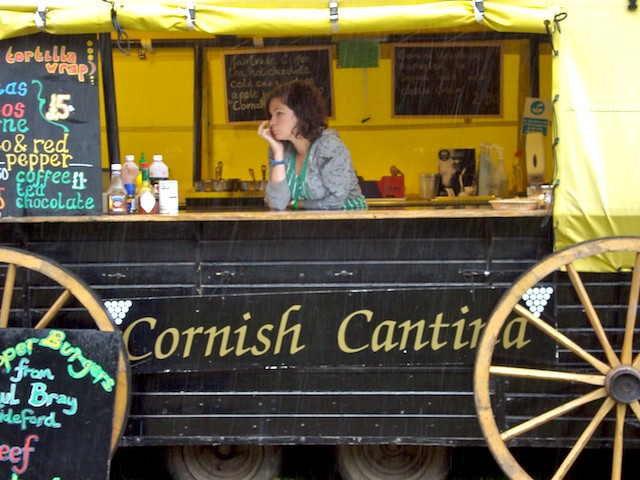The image depicts a woman standing behind the counter of a uniquely styled food truck, designed to resemble an old, two-axle wagon from the 1800s, complete with decorative wagon wheels and a train car facade. The food truck's exterior is mostly black with yellow accents, including a large black sign advertising various dishes such as "Super Burger" and "Tortilla Wrap" for $15. Some of the other menu items listed are Coffee, Tea, and Chocolate. The establishment is named "Cornish Cantina," as indicated on the side sign. The woman appears bored, resting her chin in her hand, and the scene is set on a rainy day, as evidenced by the raindrops visible in the picture.